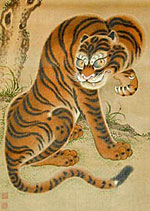The image is a traditional Japanese-style painting of a fierce-looking tiger. The tiger, depicted with black stripes on its orange body and white markings around its eyes and mouth, sits on the ground against a gold background. The tiger's deep orange nose and yellow eyes add to its intense expression, as it looks directly at the viewer. With one front paw raised and claws extended, the tiger appears to be in a gesture of intimidation or challenge. Behind the tiger, on the left side of the image, a tree with a knot hole and some grass contribute to the natural setting. The background features darker gold hues at the top, enhancing the artistic and museum-worthy quality of the illustration.